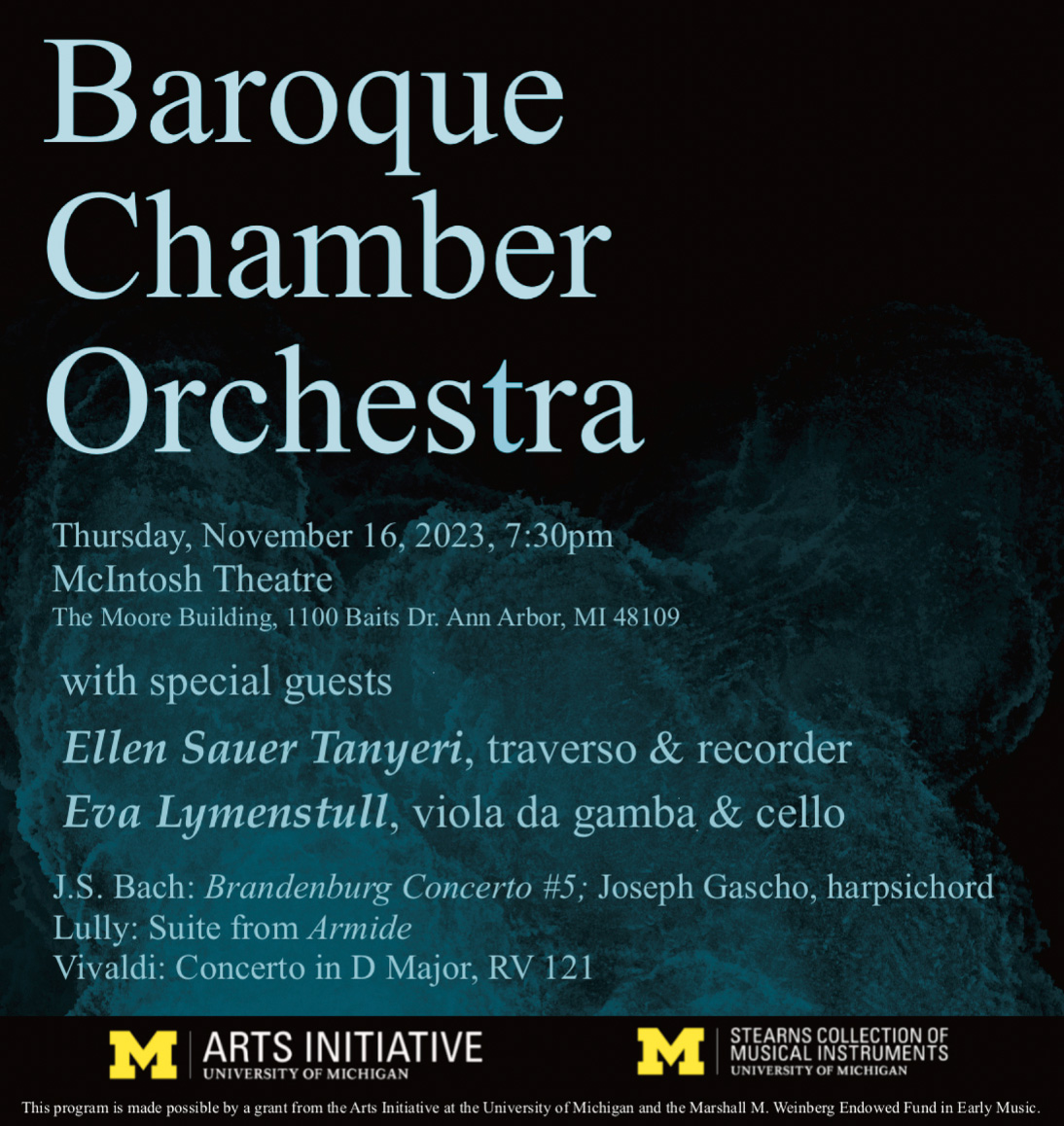Presented here is a detailed promotional graphic for the upcoming Baroque Chamber Orchestra performance. The background is primarily black with a subtle, blurred aquamarine or smoky blue gradient toward the bottom, lending a muted and atmospheric effect. The prominent large blue letters read "Baroque Chamber Orchestra." Below this, the event specifics are clearly detailed: "Thursday, November 16th, 2023, 7:30 PM at McIntosh Theater, the Moore Building, 1100 Bates Drive, Ann Arbor, Michigan, 48109."

Featured special guests include Ellen Sauer-Tannieri, who will be playing Traverso and Recorder, and Eva Limenstuhl on Viola da Gamba and Cello. The program highlights classical masterpieces such as J.S. Bach's "Brandenburg Concerto No. 5," Joseph Gascho on the Harpsichord, Lully's "Suite from Armide," and Vivaldi's "Concerto in D Major, RV121."

At the bottom of the poster, separated within a distinct black box, are the University of Michigan logos, indicating that the event is supported by the Arts Initiative and Stern’s Collection of Musical Instruments. Additionally, it states, "This program is made possible by a grant from the Arts Initiative at the University of Michigan and the Marshall M. Weinberg Endowed Fund in Early Music."